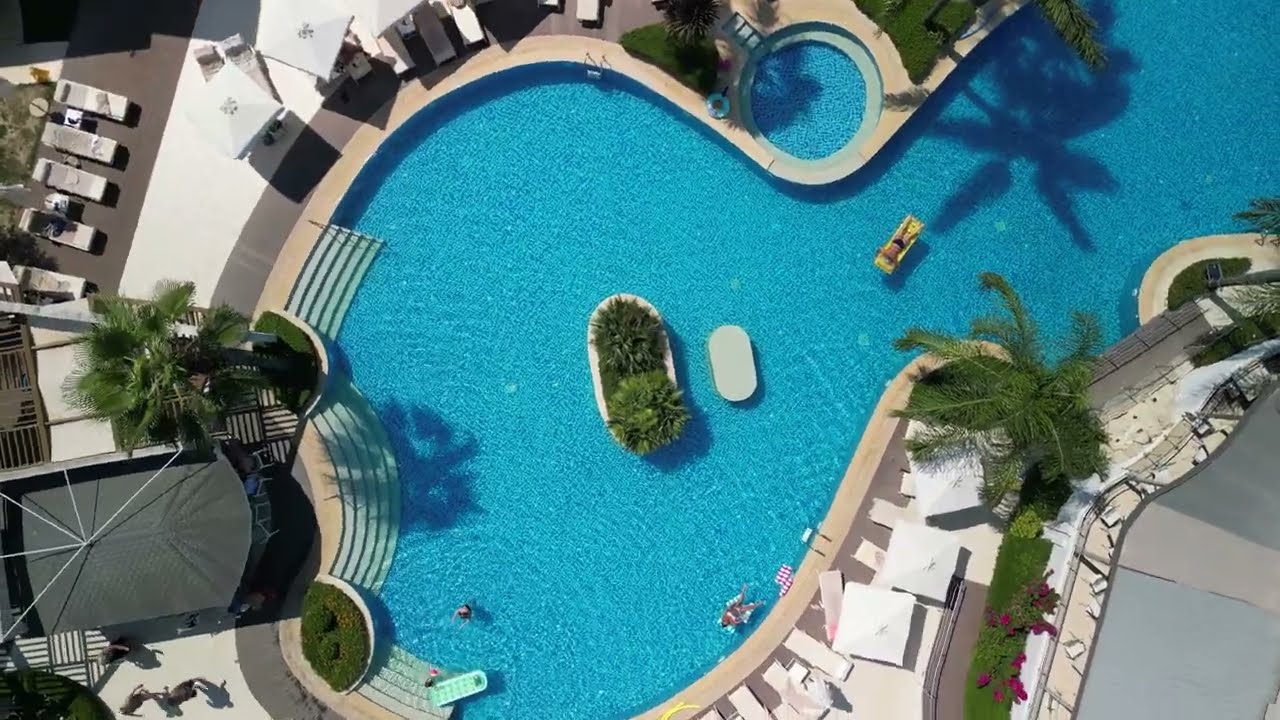This vibrant outdoor aerial photograph captures a large, uniquely shaped swimming pool, reminiscent of a spoon with its round base narrowing towards the upper right before widening again. The pool's water gleams a bright blue, likely due to the pool's blue tiling. In the pool, a man in a black swimsuit floats on a yellow rectangular floatie, while a woman reclines on a pink and white striped floatie nearby. Near the steps on the pool's left side, a few other swimmers can be seen. A small kid's pool sits atop the main pool, and an artificial island with greenery adds a tropical touch in the middle of the round area. Surrounding the pool is a spacious white deck, accented by a black stripe that mirrors the pool's curves, dotted with numerous beach chairs and white umbrellas. To the left, there's a pavilion or possibly a cafe with a black roof, while a similar gray-roofed structure sits at the bottom right. Palm trees around the pool enhance the resort-like ambiance. Scattered around the concrete deck, people walk and gather, enjoying the serene poolside environment.